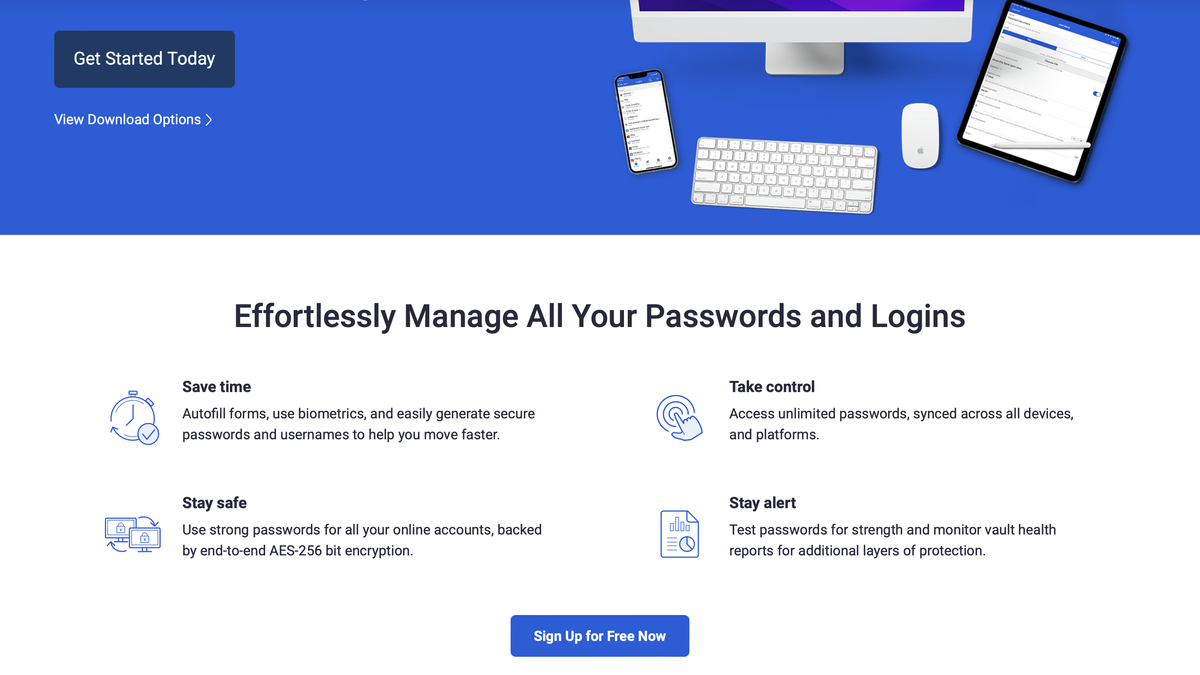Caption: 

The image is divided into two distinct halves. The bottom half features a clean, white background with prominent black text that offers detailed information about password management features. The message reads: "Effortlessly manage all your password logins." Below this are four key benefits: 

1. **Save time**: Autofill forms, use biometrics, and easily generate secure passwords and usernames to enhance your workflow.
2. **Take control**: Access unlimited password sync across all devices and platforms, ensuring seamless transitions.
3. **Stay alert**: Test password strength and monitor vault health reports for additional layers of protection.
4. **Stay safe**: Use strong passwords for all your online accounts backed by end-to-end AES256-bit encryption. 

At the bottom, a blue button invites users to "Sign up for free now."

The top half of the image contrasts with a blue background. At the top left, a call-to-action button says "Get started today," with an option below it to "View download options." On the right side, three devices are displayed: a tablet showcasing a user interface, a smartphone, and a MacBook positioned centrally, all accompanied by a white mouse and keyboard. The cohesive arrangement of devices and clean, minimalistic design reinforce the message of seamless, secure password management across multiple platforms.